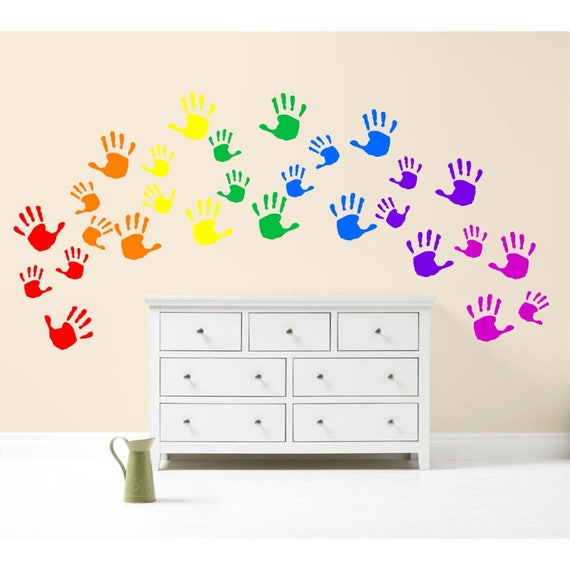This detailed photo depicts a children's artwork scene with a white dresser as the central focal point. The dresser features seven drawers, three smaller ones at the top and four larger ones beneath, accented with black knobs, and stands on a pristine white floor. In front of the dresser, there is a tall white pitcher, possibly made of stone or metal, resembling a drinking pitcher. The background showcases a peach-colored bedroom wall adorned with children's handprints arranged decoratively in a semicircle. The handprints are vividly painted in the colors of the rainbow – red, orange, yellow, green, blue, indigo, and violet – with four handprints in each color, forming a joyful, colorful arc behind the dresser.